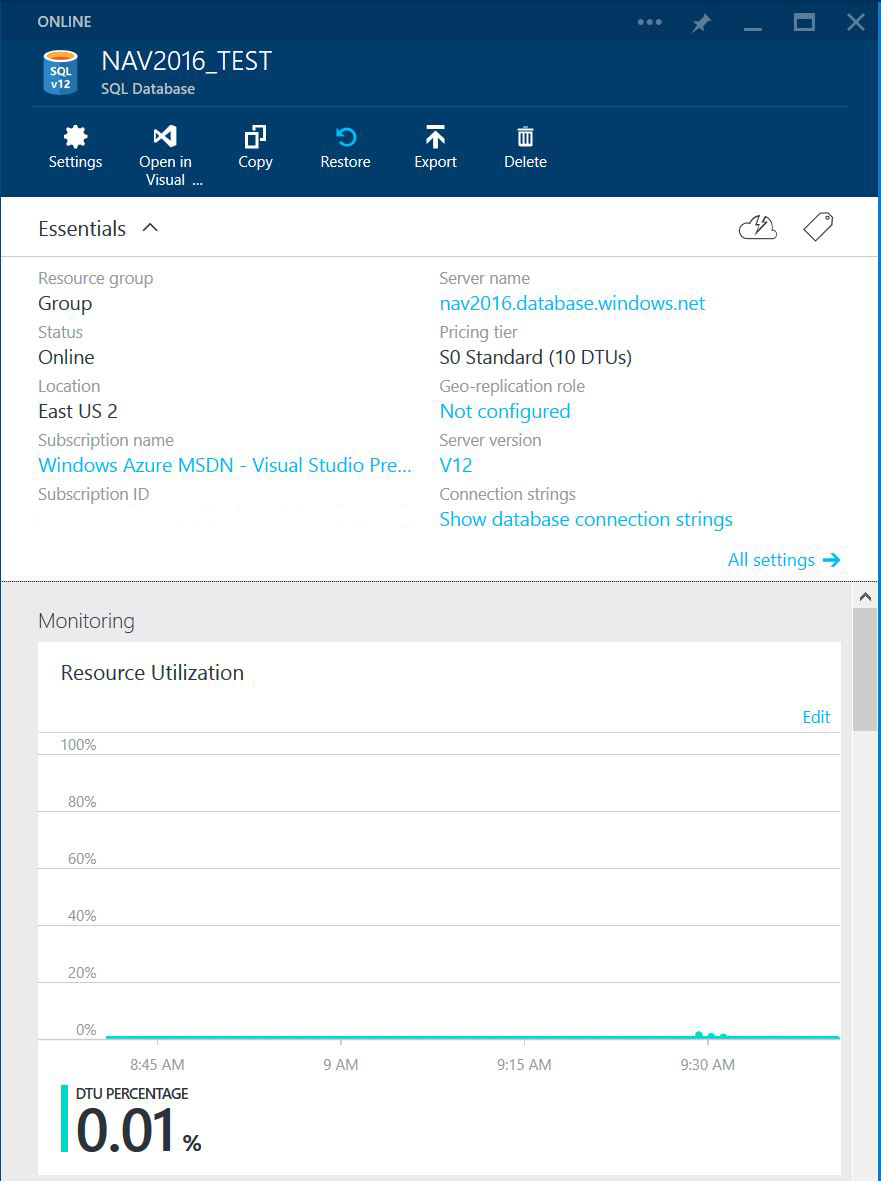This is a detailed screenshot of a website interface. The top section features a gradient background from dark blue to light blue, with a header that includes standard window controls such as the close, minimize, maximize, and pin buttons. The header text reads "online."

Immediately below the header, on a slightly lighter blue background, it identifies the SQL database with the title "NAV2016_test SQL database," accompanied by a small SQL logo and the version number "12."

Beneath this, there are various action buttons, including "Settings," "Open in Visual," "Copy," "Paste," "Restore," "Export," and "Delete."

The main content area of the screenshot has a white background. It starts with a section titled "Essentials," where the following details are listed:
- Resource Group: In Group
- Server Name: nav2016.database.windows.net
- Status: Online
- Pricing Tier: S0 Standard, 10 DTUs
- Location: East US 2
- Geo-replication: Not configured
- Subscription Name: Windows Azure MSDN Visual Studio Pre
- Version: 12
- Subscription ID: Not displayed
- Connection Strings: Show database connection strings

Following this, there is a "Monitoring" section, which shows minimal data usage with a DTU (Database Transaction Unit) percentage of 0.01%. A graph, designed to illustrate data usage from 100% down to 0%, is present but shows negligible activity. The timeline for the data displayed spans from 8:45 a.m. to 9:30 a.m., with slight variations noted around 9:30 a.m. for the 0.01% usage.

Overall, the screenshot captures a mostly static database status with minimal activity and a clean, organized layout of essential database information and action options.